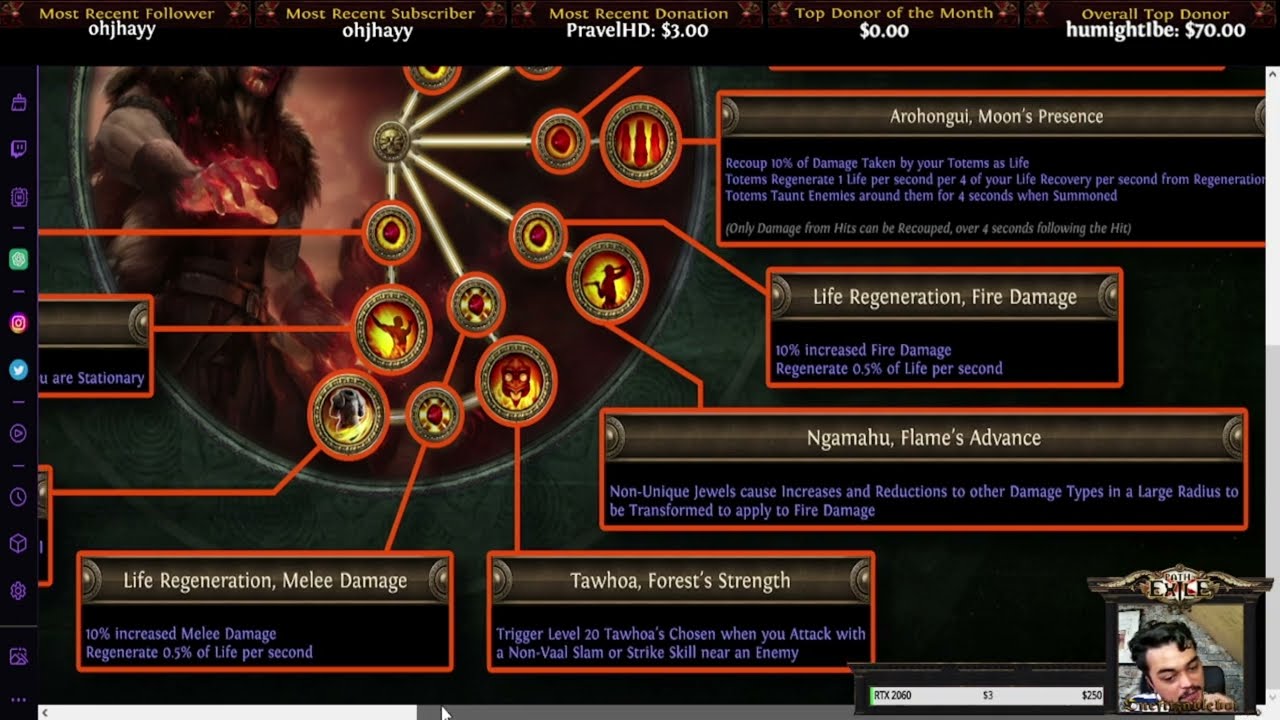The image depicts a screen from a live-streamed video game featuring an informational page loaded with various attributes and statistics. In the bottom right corner, there is a webcam feed of the streamer, showing a man's face labeled "With Exile." The top portion of the screen is dominated by a banner displaying donation and subscription stats, including "Most Recent Follower" and "Most Recent Subscriber" listed as OHJHAYY, "Most Recent Donation" by Praval HD of $3, "Top Donor of the Month" showing $0, and an "Overall Top Donor" with a contribution of $70.

The central and left portions of the screen are adorned with numerous pendants bearing distinct images, likely signifying various capabilities within the game. These items are organized in a grid layout centralized around a core circle. Each pendant has accompanying text that details specific attributes, including "Aura Hungle Moon's Presence," "Life Regeneration," "Fire Damage," "NGA Mahou Flames Advance," "Tahoa Spore Strength," and "Melee Damage." The color scheme is rich with dark, fiery hues like reds, yellows, and browns, accented by darker slate tones, contributing to the game's mythical ambiance.

In the top left, a creature with a fiery hand commands attention, suggesting a character or adversary within the game. Various social media icons, including those for Twitch, Instagram, and Twitter, are arranged vertically like a menu bar, presumably providing quick access links for the audience. Lines connect the informational text bubbles to their respective icons or imagery, ensuring a detailed and visually engaging display for viewers following along with the stream.